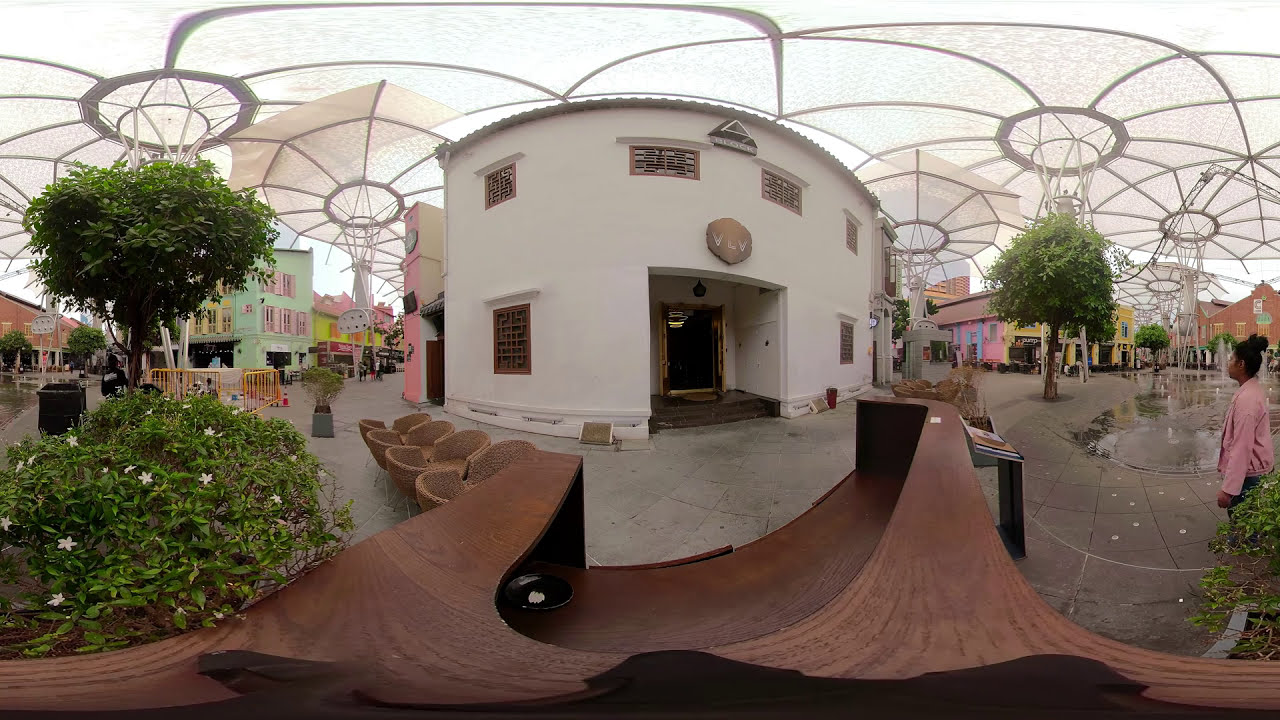In this panoramic image of an outdoor area, the focal point is a round, white stucco building with a flat roof and beige trim. Above the entryway is a distinctive wooden plaque with a "VV" symbol. The building features windows adorned with intricate wooden designs. The foreground of the image showcases a series of brown lines that are part of a seating area made from a carved wooden log. Surrounding the building are sheer canopies made from white or silver wires. To the left, a topiary tree and a green bush with white flowers can be observed, while the right side features another topiary tree and additional shrubbery. A woman in a pink long-sleeve shirt stands on the right side of the image, looking towards the building. The background includes several colorful buildings—light green, yellow, pink, and brick red—suggesting a vibrant, possibly commercial or mall setting. The canopies are not continuous, allowing light to filter through in certain areas.